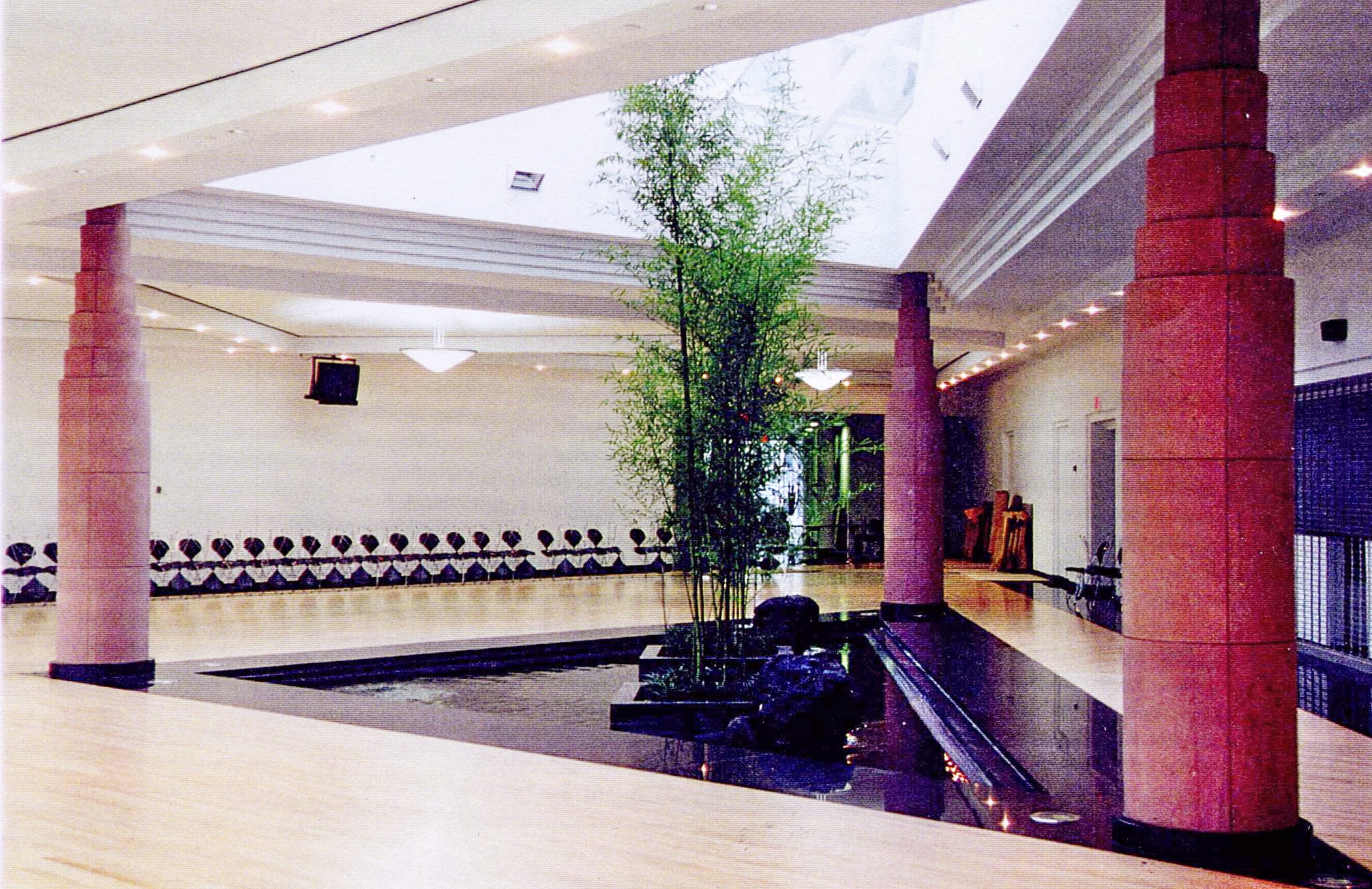This image, likely a photographic projection onto a textured surface such as cloth or paper, depicts the interior of a spacious building that could be part of a mall or museum. The focal point is a triangular atrium with a skylight shaped similarly, allowing sunlight to illuminate a central fountain containing planters with tall, skinny trees. The area is bordered by columns—three prominently red-toned pillars with a telescoping, layered design, forming a triangular pattern themselves. The flooring around the fountain is wooden, featuring a thick black stripe that mirrors the triangle's shape. The backdrop includes white brick walls adorned with a unique design of black wave patterns and circles along the bottom. Additional details include a gated storefront to the right, possibly indicating a closed shop or exhibit, and various lighting elements around the perimeter. On the ceiling's left side, a monitor is visible, while the right side features a blue wall, contributing to the overall aesthetic of the muted, slightly desaturated, soft-toned image.